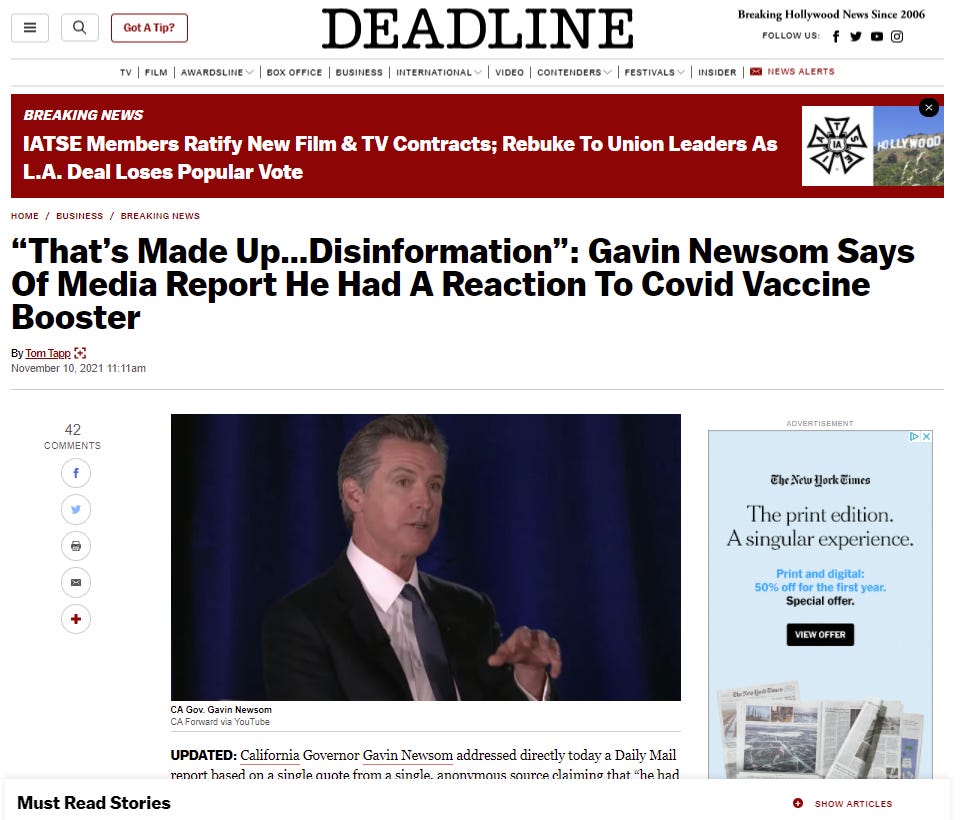This image is a cover page of the newspaper "Deadline" from the Breaking Hollywood News source, established in 2006. The search bar on the cover features "Got a tip?" in red. The primary headline reads, "Breaking News: IATSE members ratify new film and TV contracts, rebuke to union leaders as LA deal loses popular vote." Below this headline, there is a subheading that reads, "Disinformation: Gavin Newsom says of media report," referring to misinformation regarding his reaction to a COVID vaccine booster. 

The cover includes a photograph of California Governor Gavin Newsom, accompanied by the caption, "Updated: California Governor Gavin Newsom addressed directly today a Daily Mail report based on a single quote from a single anonymous source claims that he had..." (the text cuts off here).

The page shows that there are 42 comments and features social media icons for Facebook, Twitter, and three other platforms. Adjacent to the social media section, there is an advertisement for The New York Times, promoting a special offer for their print and digital editions with the text, "A singular experience, print and digital, 50% off for the first year. View offers."

This detailed description captures the essence of the "Deadline" cover page.